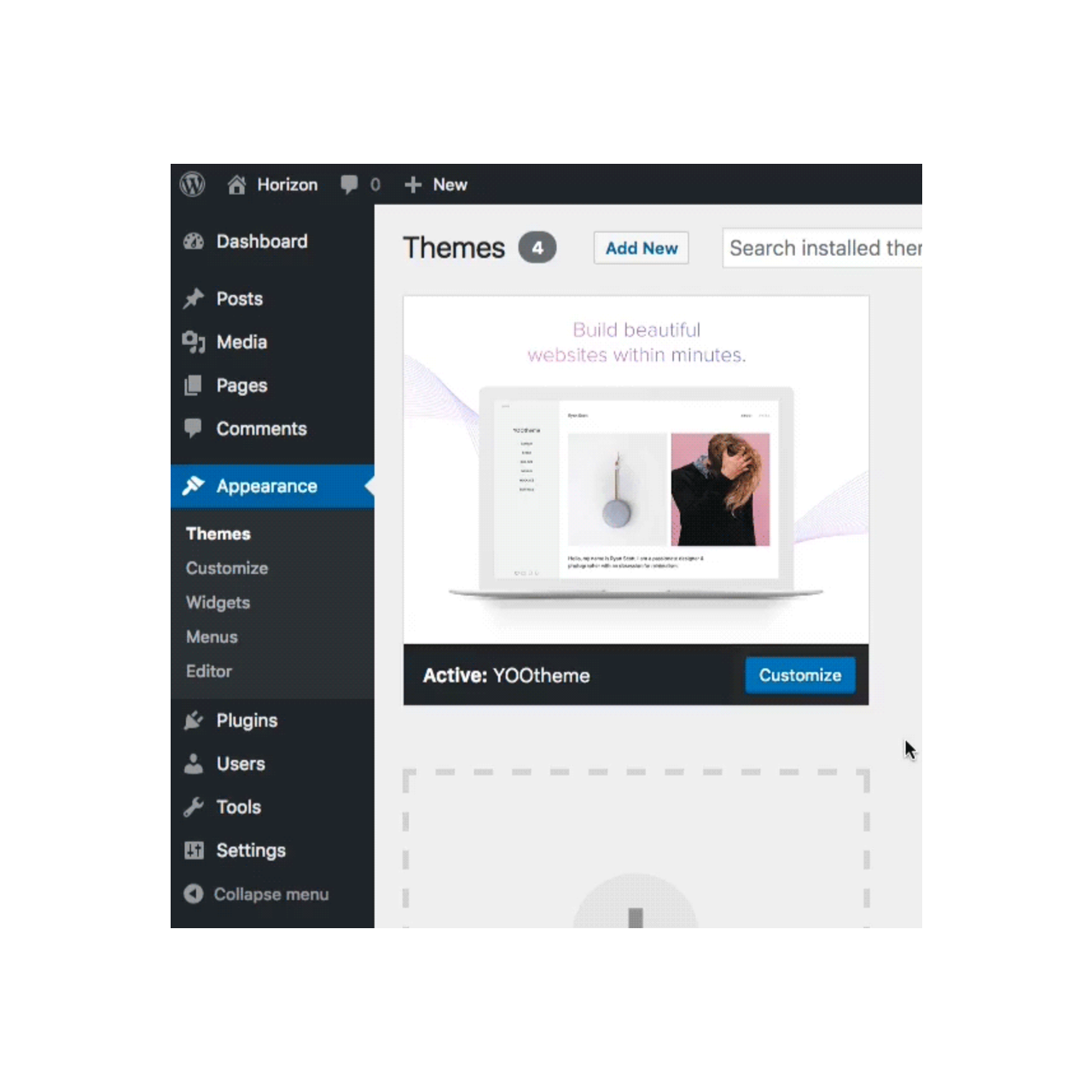This image is a screenshot from a computer interface, likely a content management system. The interface features a black sidebar on the left and a black menu bar along the top, both filled with white text. In the top left corner, there is a logo, next to which is a house icon labeled "Horizon." Next to that, there is a text bubble icon with the number zero beside it, followed by a plus sign and the word "New."

Down the left sidebar, categories are listed as follows: Dashboard, Posts, Media, Pages, Comments, Appearance (which is highlighted in blue), Themes, Customize, Widgets, Menus, Editor, Plugins, Users, Tools, Settings, and Collapse Menu. The blue highlighting indicates that the Appearance category is currently active, showing its options on the right side of the screen.

In the main content area on the right, there is a header that reads "Themes 4" with an "Add New" button nearby. Another button labeled "Search Installed" is partially visible. Below, a background image displays a template preview with the text "Build Beautiful Websites Within Minutes." The template is identified as "Active YOO Theme," and there is a blue "Customize" button beneath this text. Lower in the interface, a dotted line square contains what appears to be a circle with a plus sign in the middle, though the plus sign is not fully discernible.